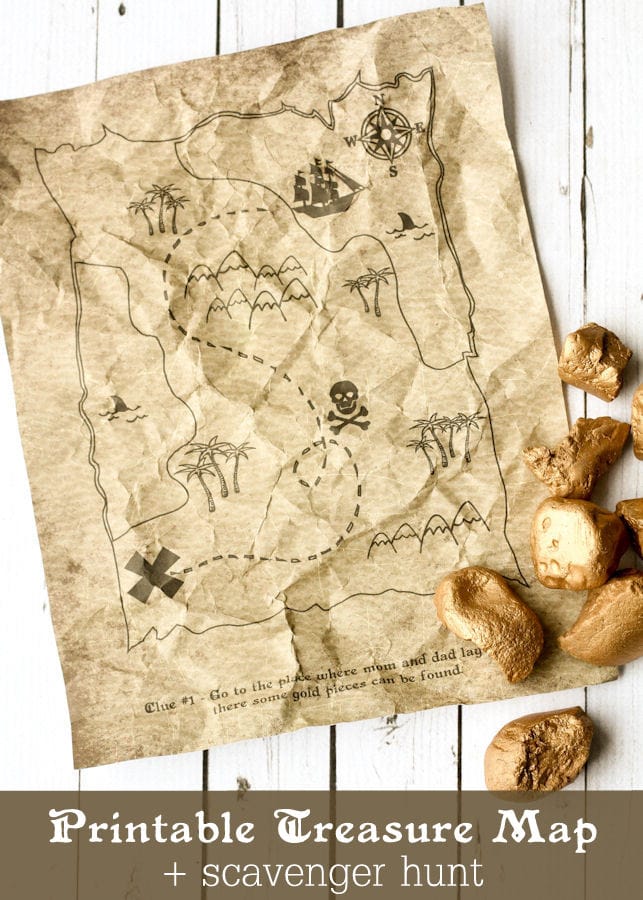This image is a photograph of a weathered, crumpled treasure map laid on a white wooden table. The map, labeled at the bottom under a transparent brown rectangle with the words "printable treasure map + scavenger hunt," features a detailed route marked by a dotted line. The line winds through various illustrations, including trees, mountains, a skull and crossbones area, and swirls, eventually leading to a large X at the lower left corner. A compass rose indicating North, East, South, and West is depicted at the top alongside a ship, while two sharks' fins appear in the water sections on both the top and left sides of the map. The map is held down by objects meant to resemble gold pieces or brown rocks, especially noticeable in the lower right corner. An additional note at the bottom of the map reads, "Clue number one, go to the place where mom and dad lay. There, some gold pieces can be found."